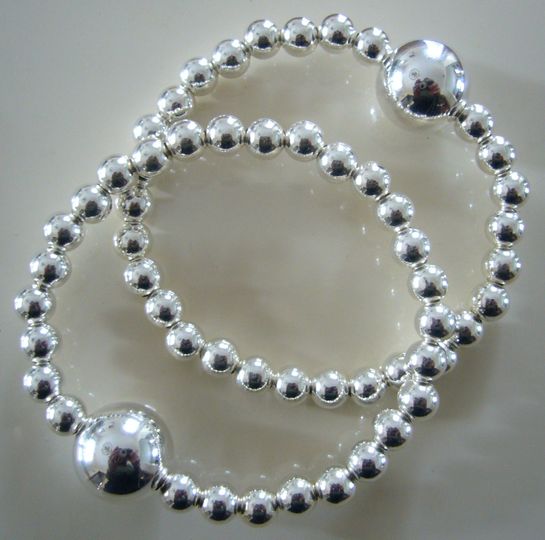The image showcases two intricately designed silver wristbands, each composed of multiple small, highly reflective silver spheres arranged in a pearl bracelet style. These spheres uniformly encircle each wristband, culminating in a single, significantly larger sphere at one end of each piece. The wristbands are meticulously stacked in a diagonal arrangement, with one extending from the bottom left to the top right, and the other from the top right to the bottom left, against what appears to be an off-white, shiny surface. The reflective quality of the silver spheres is so pronounced that you can discern the image of the photographer taking the picture in each one. The captured setting, likely a jewelry store or home collection, casts delicate shadows that add depth to the image. The striking symmetry and glossy finish of the wristbands, coupled with their detailed reflections, create an elegant, visually captivating composition.